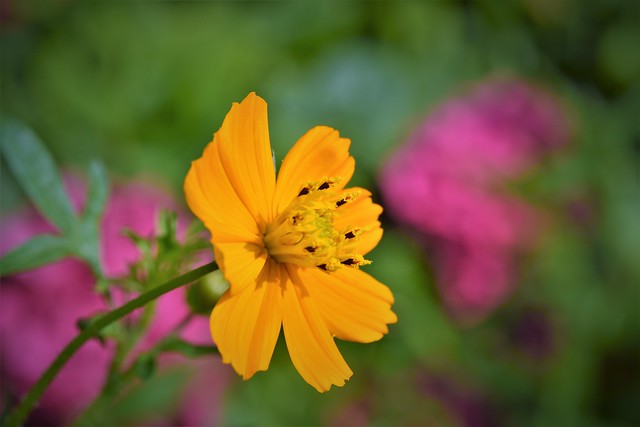This image showcases a vibrant, orange-yellow flower, possibly a cosmos, in full bloom at the center of the frame. The flower, which has about eight petals with a few separations, displays intricate details including visible stems, petals, and lines, with a green pistil emerging from its center. Surrounding the focal flower, out of focus, are two large pinkish-purple flowers flanking either side, hinting at a colorful background. Further in the background, blurred green vegetation adds a contrasting backdrop, emphasizing the central flower's bright, detailed appearance. The overall composition and shallow depth of field highlight the central flower's vivid hues and sharp details against the softer, indistinct greenery and additional blossoms.